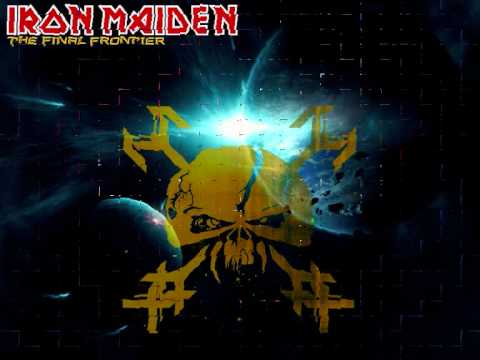This detailed image depicts what appears to be a poster or album cover for the heavy metal band Iron Maiden. Prominently featured in the upper left corner, the band's name "Iron Maiden" is displayed in bold red text outlined in white, with "The Final Frontier" written below in smaller yellow letters. The central artwork showcases a vividly illustrated yellow skull with angry, angular eyes and prominent fangs, giving it an alien-like appearance. This menacing skull seems to be floating in outer space, surrounded by elements that underscore the cosmic theme—a dark expanse dotted with planets and a radiant star emanating pale blue and white light from the center. One larger, more detailed planet is situated at the top right corner, while a smaller one is towards the bottom left. The overall dimensions of the image are slightly wider than taller, suggesting it could be a promotional poster rather than a traditional album cover. Intricate lines with branching patterns extend from the diagonal corners of the skull, further adding to the otherworldly and highly detailed nature of the artwork.